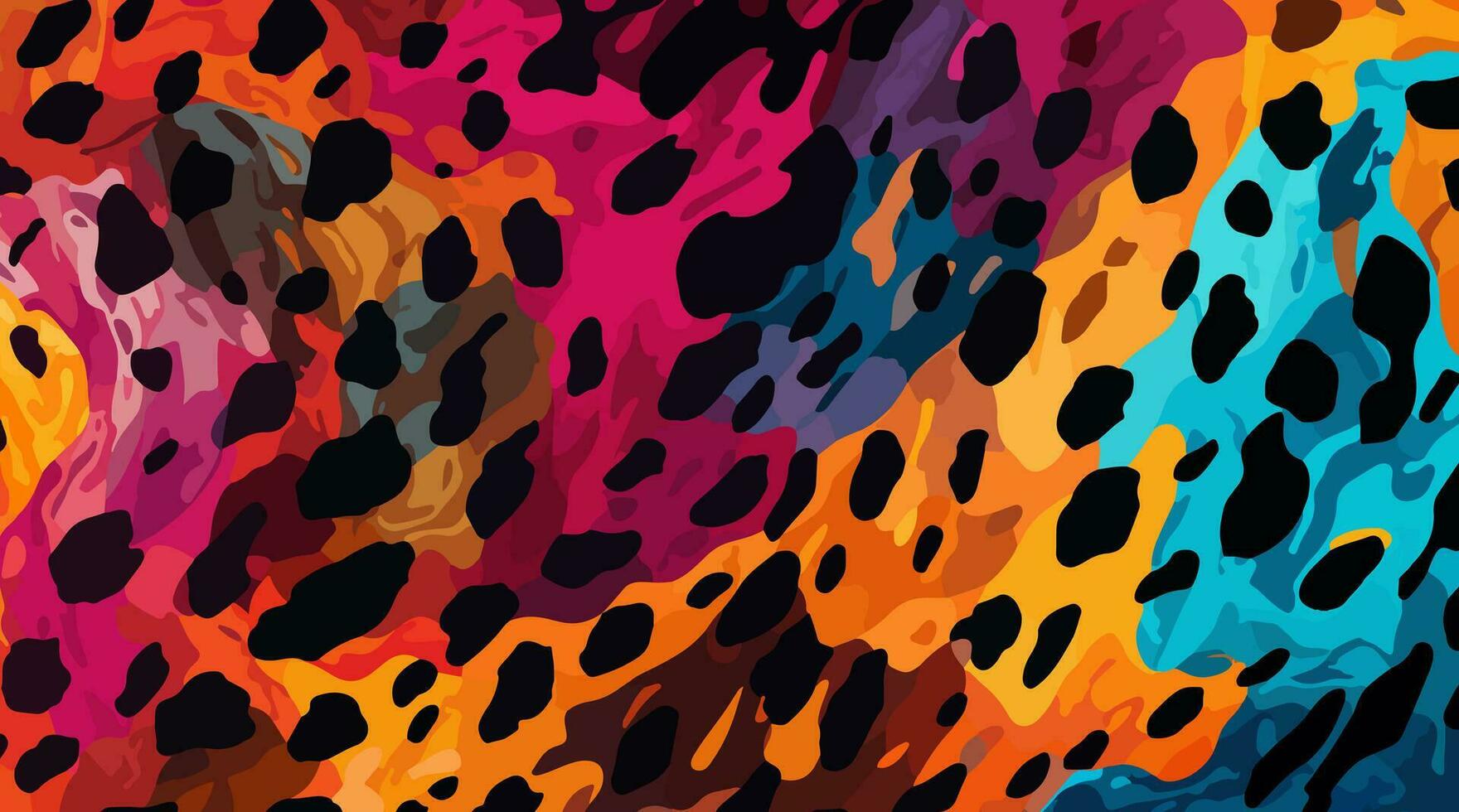This is a vivid and dynamic painting or illustration in a horizontal rectangular orientation. The artwork features an intricate array of amorphous and overlapping shapes in a riot of colors, including bright blue, hot pink, orange, brown, red, yellow, and gray. These shapes fill the entire background, with no white space remaining, creating a rich tapestry of color interactions. Overlaying this colorful backdrop are irregular, jaguar-like black spots that add a striking contrast and pattern to the composition. The overlapping colors often blend to form new shades, such as purple where pink and blue meet, creating an imaginative and eye-catching effect. Though complex in its interplay of colors and patterns, the overall abstraction suggests both a sense of chaos and harmony.